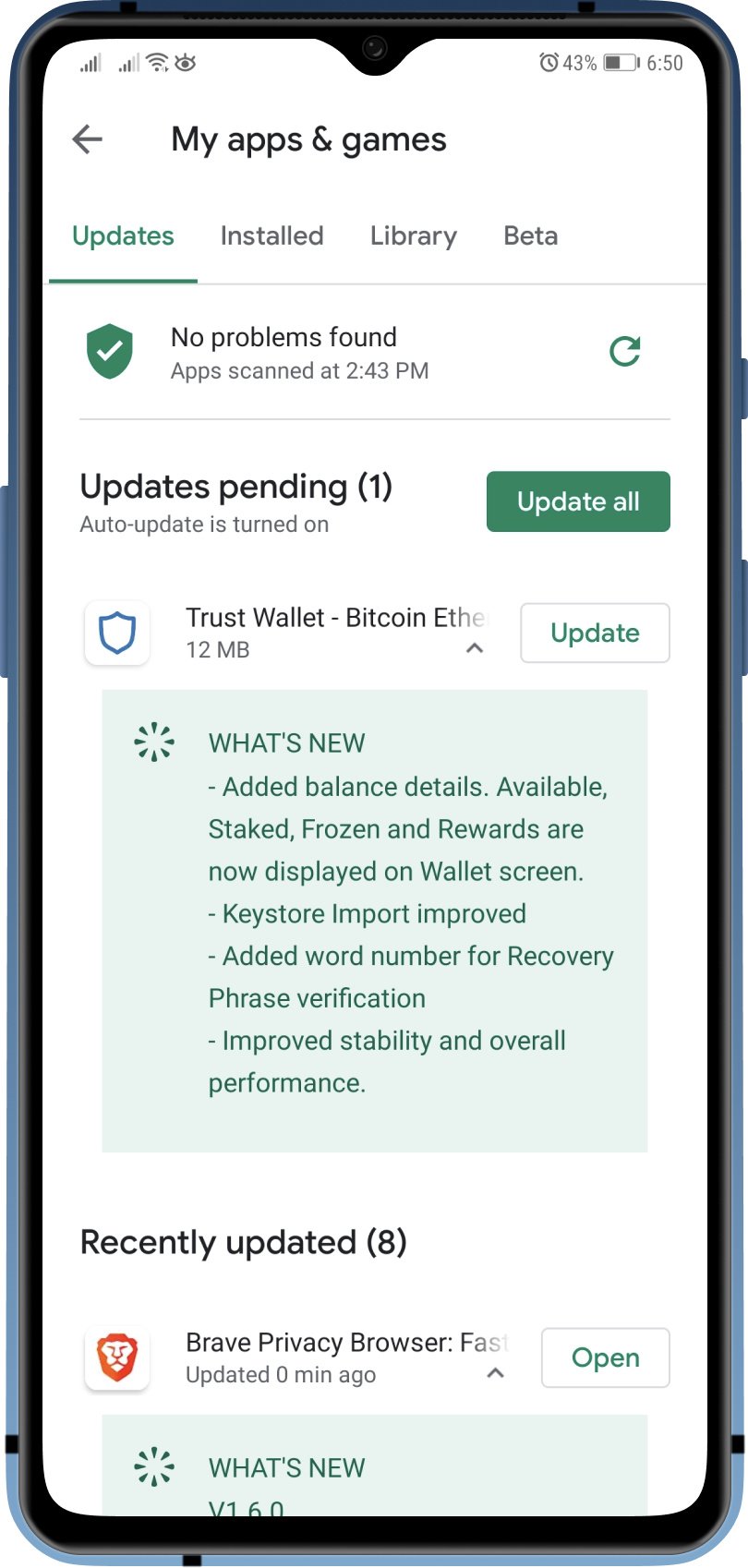This image is a detailed digital photograph of a mobile phone's screen, showcasing the "My Apps & Games" section of an app store interface. The phone's frame and buttons are visible, providing context to the displayed content. The screen prominently features a white background.

At the top of the screen, the title "My Apps & Games" is clearly visible. Below this title, there are four tabs, with the "Updates" tab highlighted in green. To the right of "Updates," additional tabs labeled "Installed," "Library," and "Beta" are aligned.

Directly beneath these tabs, a banner displays a green shield with a white check mark accompanied by the message "No Problems Found. App scanned at 2:43 PM."

Following this banner is a section marked "Updates pending (1)," alongside a prominent green "Update All" button. Below this, the screen shows a single pending update for the app "Trust: Crypto & Bitcoin Wallet," identifiable by its icon featuring a white background with a blue shield.

A light green box accompanied by dark green text details the changelog for this app, listing updates such as "Added Balance Details," "Key Store Import Improved," "Added Word Number for Recovery Phrase Verification," and enhancements in "Stability and Overall Performance."

At the bottom of the screen, a header labeled "Recently updated (8)" introduces the recently updated apps section. The first and only visible recently updated app is "Brave Private Web Browser," identifiable by its icon of an orange lion set against a white background.

This descriptive caption provides a thorough visual and contextual understanding of the mobile phone screen's interface and the specific details it displays.